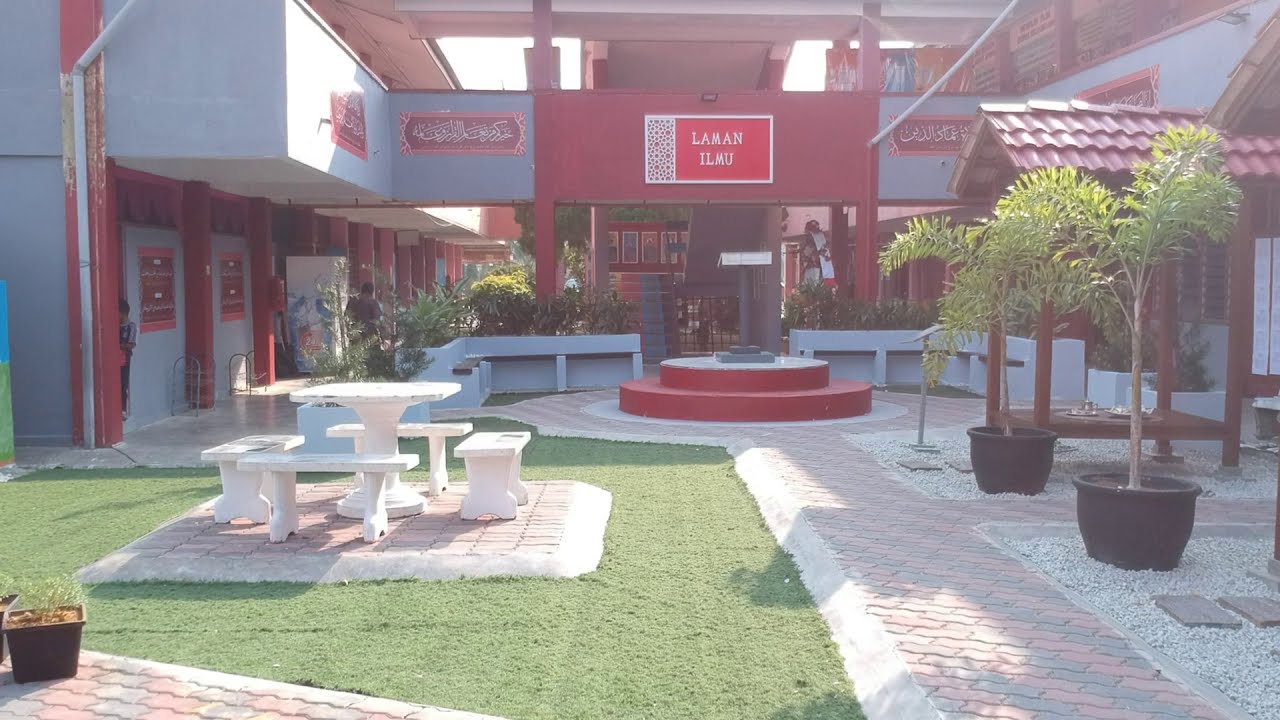In this daytime image of a courtyard, we are situated in front of a large building complex that appears to be a restaurant or shopping district. The two-story building features gray walls with prominent red support beams and posts. A key focal point in the center of the courtyard is a red-bricked, round two-step foundation with a podium or structure on top of it. A cobblestone pathway runs down the center, flanked on the right by gravel with multiple black pots containing small green trees or fern-like plants.

On the left side of the walkway, there is a lush green lawn area with a square cobblestone section. Positioned on top of this square is a white stone table surrounded by four matching white stone benches. Details such as gray pebbles on the ground and various signs, including a notable red sign with white writing spelling "L-A-M-A-N-I-L-M-U," enhance the bustling and organized ambiance of this commercial or dining area.